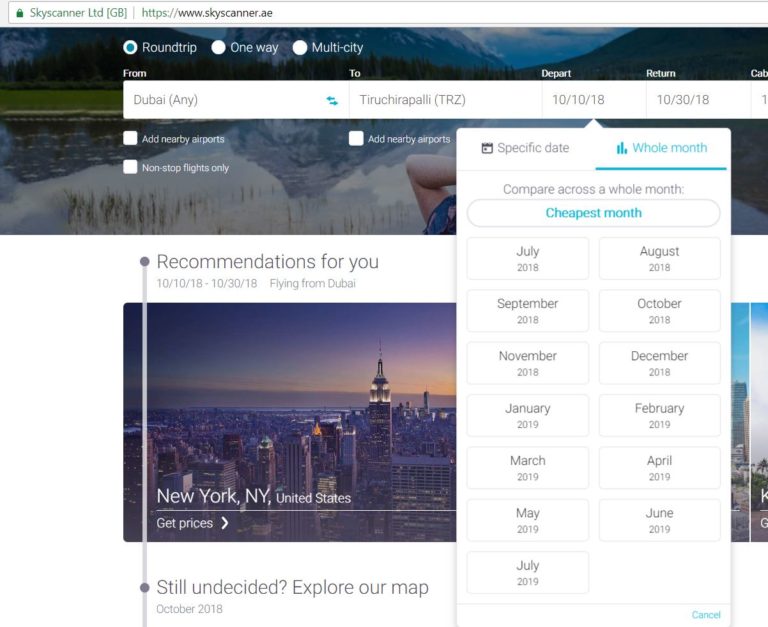The Skyscanner Ltd website offers a comprehensive tool for comparing airline ticket prices. At the top of the page, there is a stunning photograph showcasing a mountainous region, with tall alpine trees and a large, serene lake in the background. Below the photograph, users are presented with three travel options in a form: "Round-Trip" (highlighted), "One-Way," and "Multi-City." 

In the form fields, Dubai (origin) and Tiruchirappalli TRZ (destination) have been entered, with departure and return dates set for October 10, 2018, and October 30, 2018, respectively. Just beneath the form, text provides personalized recommendations, stating "Recommendations for you flying from Dubai." Accompanying this text is an enticing picture of New York, New York, United States. Additionally, a message encouraging further exploration reads, "Still undecided? Explore our map."